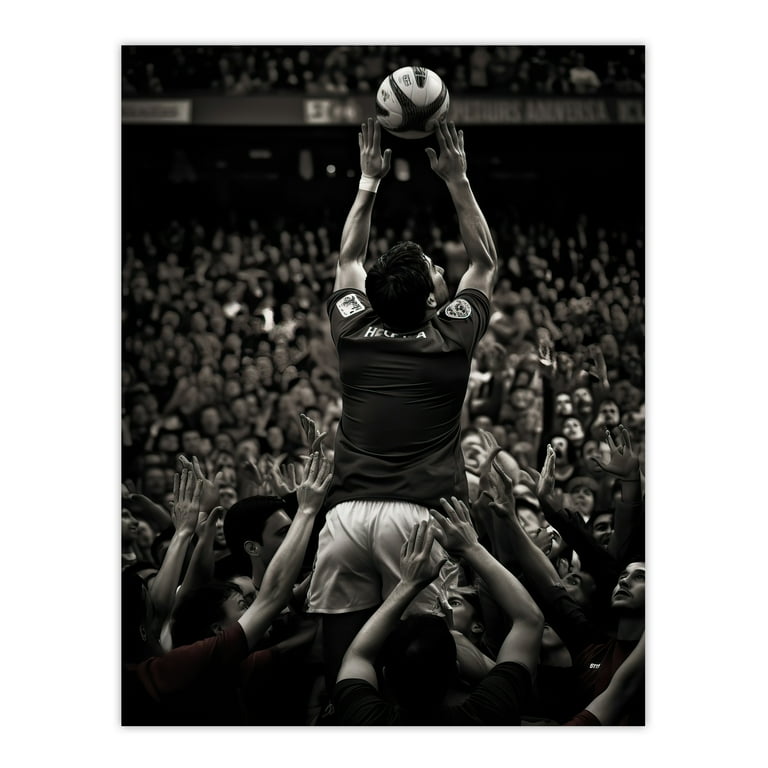This black-and-white photograph captures an intense sports scene in a packed stadium. The top two-thirds of the image displays a blurred crowd of seated spectators, with the stripe of the stadium mezzanine visible near the top. The bottom third is dominated by a dense crowd of people, all reaching their bare arms upwards, creating a dynamic sea of hands. At the center of the frame, a man with short hair is airborne, wearing short, glossy white shorts and a wide, black short-sleeve jersey adorned with two emblems on the shoulders— a white rectangle with a black design on the left and a white teardrop shape with a black design on the right. His left wrist sports a white band, and he is looking up and to the right with his fingers fully extended towards a ball in midair. The ball, likely a soccer or rugby ball, is mostly white with a distinctive black X shape across the front and two black tendrils—one on the top and one to the left. Surrounding him, a multitude of people, seemingly all men, also have their hands lifted in the air. The background suggests a large venue filled with advertisements that hint at a giant stadium setting. The photograph exudes a sense of high energy and anticipation, capturing a pivotal moment in the game.